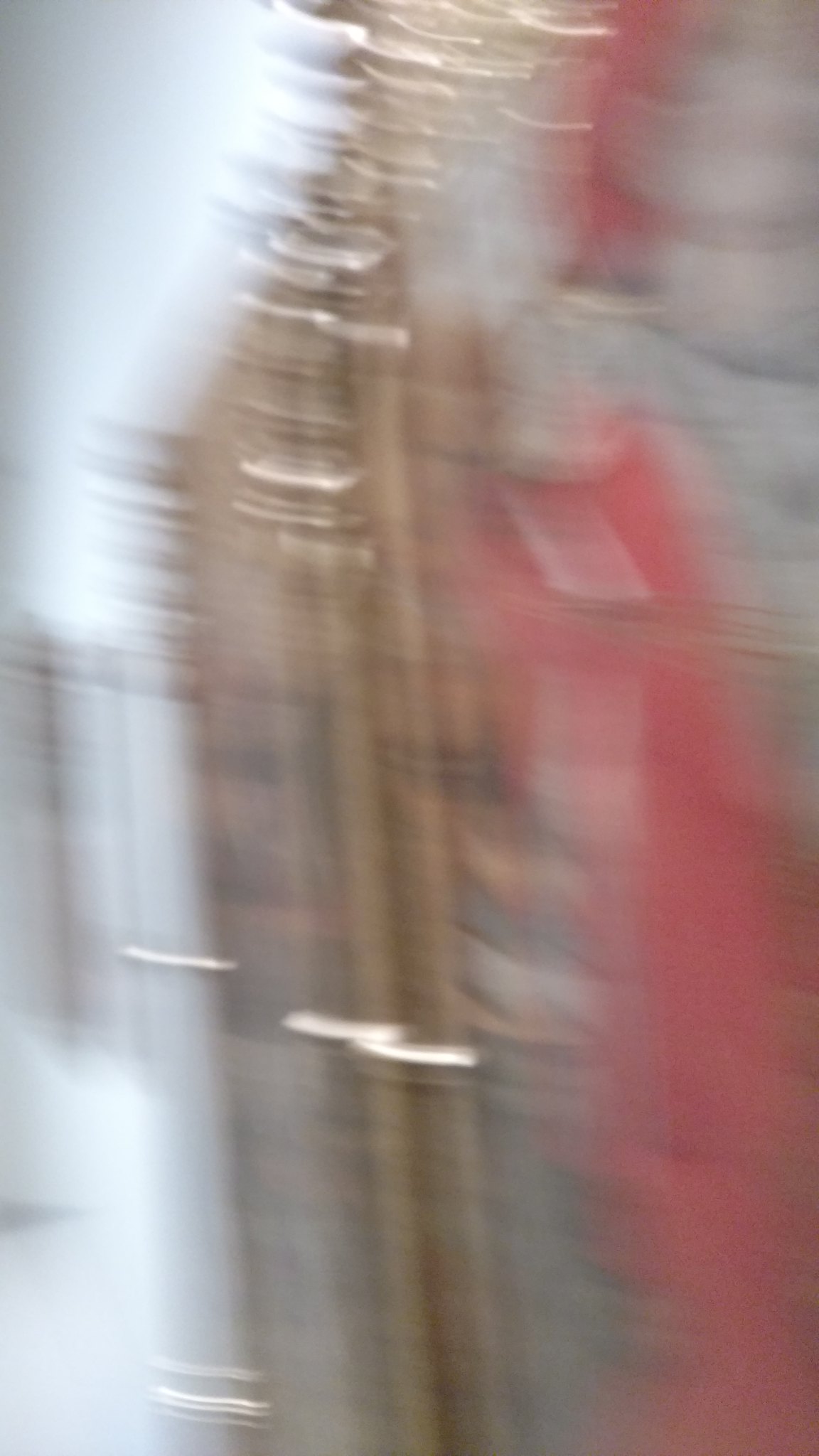This extremely blurry photo captures a scene that is difficult to identify clearly due to the lack of focus, perhaps caused by camera movement or a shaking hand. Central to the image is a metallic structure that appears to be golden, resembling bars or a frame. This golden element could be part of a larger object, such as a door, a mirror, or an instrument. The golden structure seems to feature smaller, additional pieces at the top and possibly silver handles, adding to its complex appearance.

The background includes various color patches: shades of white and gray dominate the scene, providing some sort of backdrop. On the right side, there is a prominent red structure that stands out but remains indistinct due to the blurriness. The area's top right corner also includes something white, adding to the color variety. Certain dark (perhaps black) rectangles or strips blend into the scene, making it even more perplexing to determine any specific details.

Overall, the image contains a blend of gold, white, gray, and red colors, set against a gray and white background, with elements that might be architectural or ornamental. The photograph's composition, taken from a side angle, adds to the difficulty in identifying the objects within.